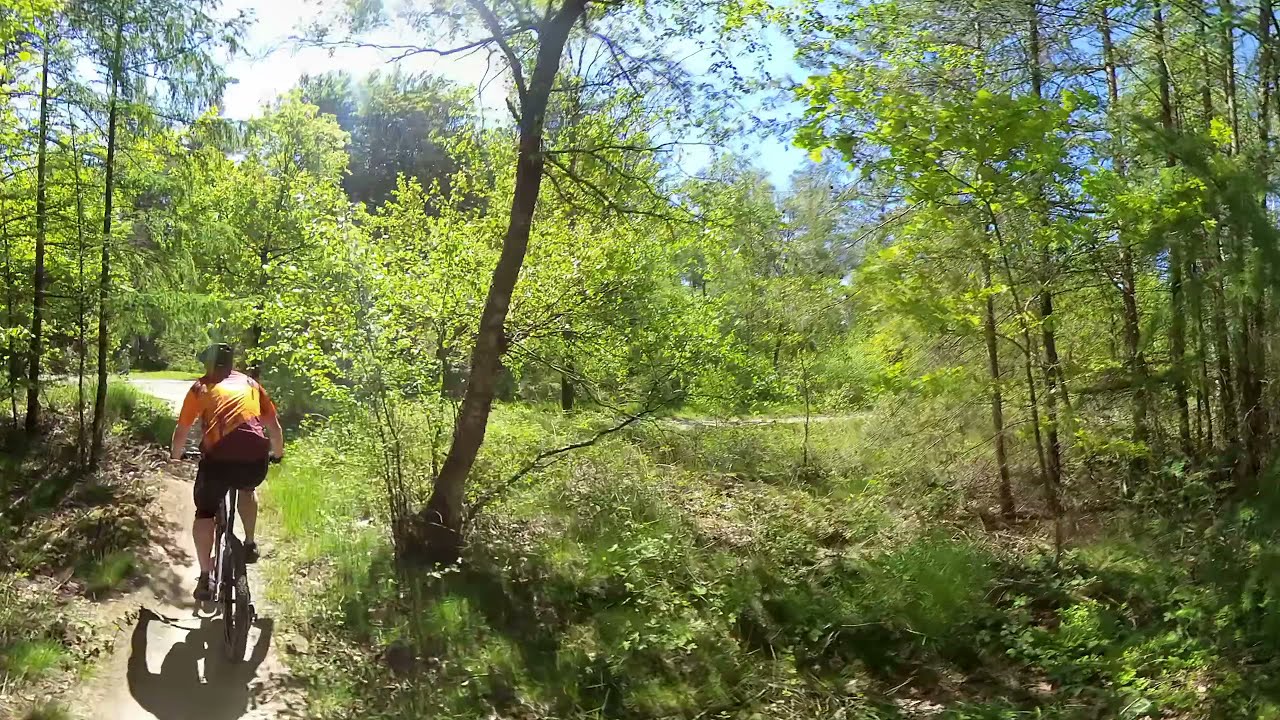This landscape-oriented photograph captures a tranquil outdoor scene of a solitary bicyclist riding down a narrow dirt trail that meanders through a wooded area. The trail, which appears suitable for either hiking or biking, can be seen on the left side of the image before veering to the right behind some brush at the midline. The rider, facing away from the camera, sports a short-sleeve shirt with orange and yellow hues, black knee-length shorts, black and white socks, and black shoes. Topping off the outfit is a black helmet, ensuring safety as they navigate the path. The surrounding environment is lush with tall trees in various stages of fall foliage, dense underbrush, and an open, sloping area to the left suggesting a hillside. The sky above is a mix of blue with scattered white clouds, indicating a sunny day. The combination of thriving greenery and hints at a past or distant stream add to the naturalistic charm of the scene.